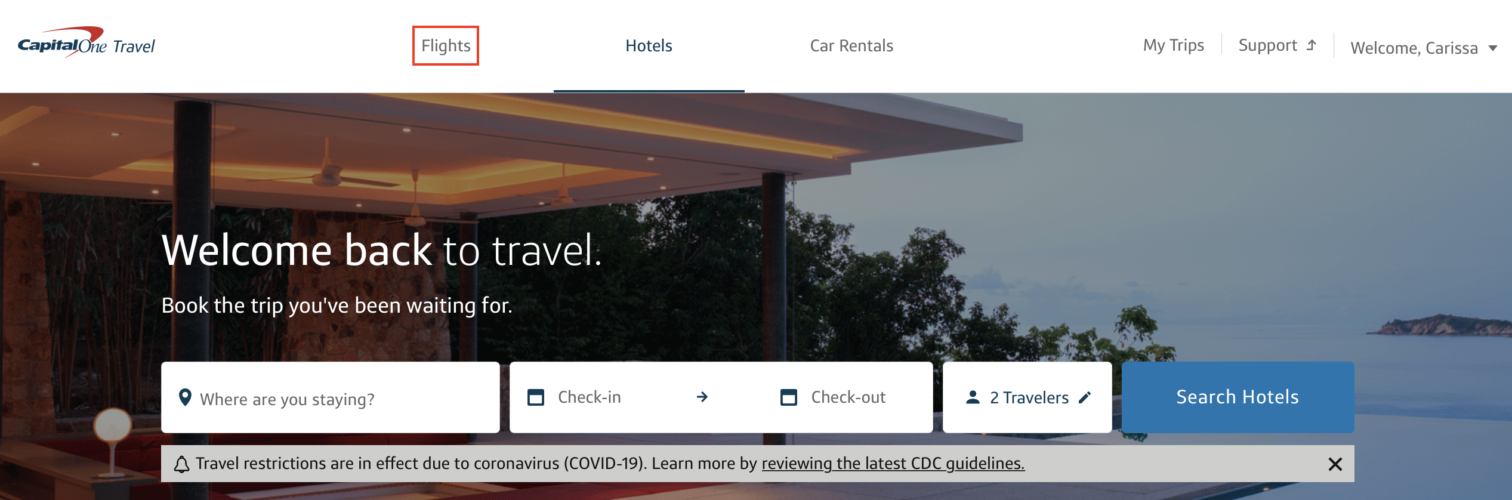Here is a detailed and cleaned-up caption for the image:

---

A cropped screenshot of the Capital One Travel website features the upper section of the page. At the top left, the Capital One Travel logo is prominently displayed. Centralized in the header are three navigational categories: "Flights," "Hotels," and "Car Rentals." The "Flights" category is emphasized with an edited red box around it, while "Hotels" is currently selected, indicated by a blue underline beneath it. Below this header bar, the background transitions to a welcoming image with text overlay. On the left side, bold white text reads, "Welcome back to travel," followed by a smaller, encouraging message below: "Book the trip you've been waiting for." Beneath this, a search functionality is displayed. It includes a main search bar, with adjacent check-in and check-out date fields to its right. Further right, there's a "Travelers" option box and a blue "Search Hotels" button for initiating the search. An informational banner across the bottom highlights ongoing travel restrictions due to COVID-19, advising users to "Learn more by reviewing the latest CDC guidelines." An 'X' icon is positioned on the right of this alert banner, allowing users to dismiss the notification.